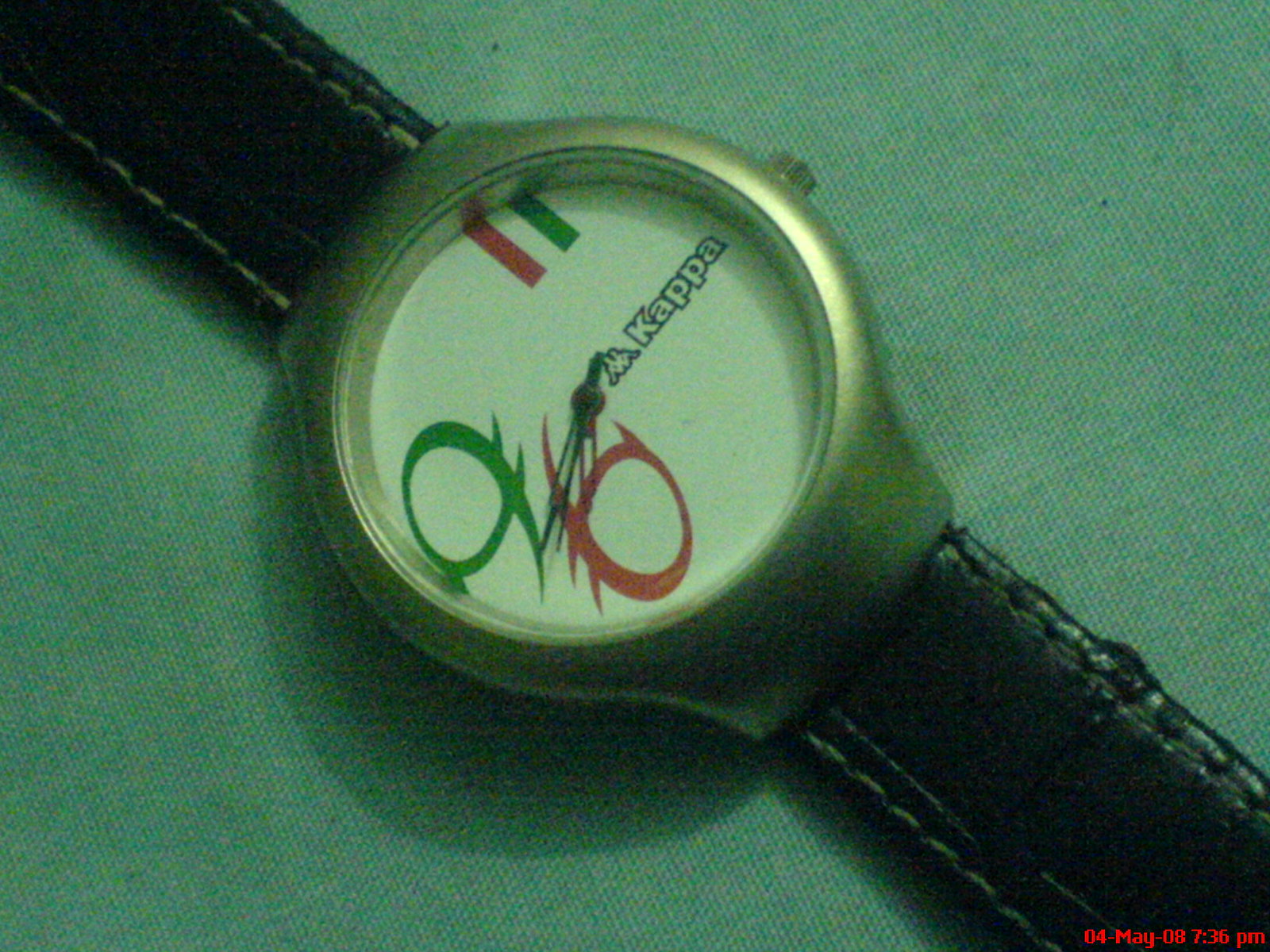This image captures a Kappa brand wristwatch meticulously placed on a white, cotton-like fabric, enhancing its elegance. The texture of the fabric and its delicate folds are subtly visible, though tinged with a greenish hue due to an apparent filter, giving the whole photograph a unique, vintage feel. The photo itself has a grainy quality, adding a layer of rustic charm to the overall composition.

The focal point, the Kappa watch, prominently features the iconic logo of two figures sitting back-to-back. The watch’s dial is minimalist yet striking, with large numerals: a prominent "9" at the nine o'clock position and a slightly shifted "6" at the six o'clock position. The design is accented by small spikes on the sides of the numbers, adding a touch of edginess. A distinctive red, yellow, and green rectangular flag adorns the top of the dial, adding a splash of color and cultural flair. The use of green and red designs further embellishes the watch face, making it not just a timepiece but a statement accessory.